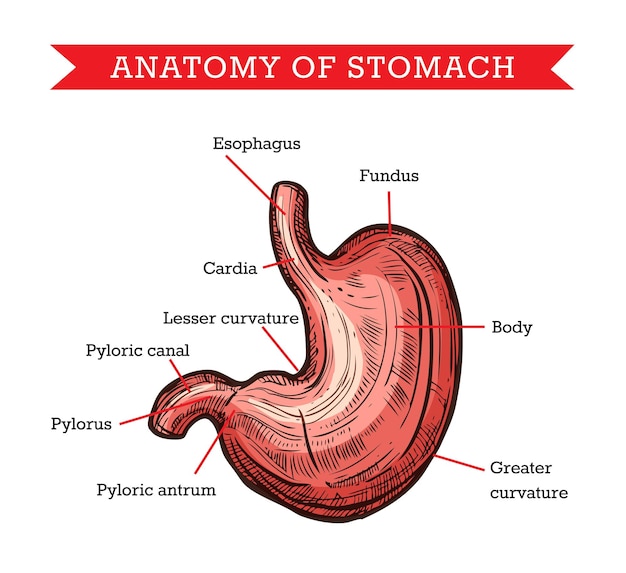The image is a detailed, color illustration of the anatomy of the stomach, prominently featuring a curved, reddish organ with various parts labeled. At the top, a red banner with white text reads "Anatomy of Stomach." The illustration shows the stomach in shades of red, pink, and cream, with black text labeling each section. Labels identify the major parts including the esophagus at the top, the fundus, the body, and the greater curvature. To the left, the pyloric antrum, pylorus, and pyloric canal are marked, while the lesser curvature and cardia are also indicated. The drawing includes numerous black lines to add texture and detail, giving a comprehensive view of the stomach's anatomy.